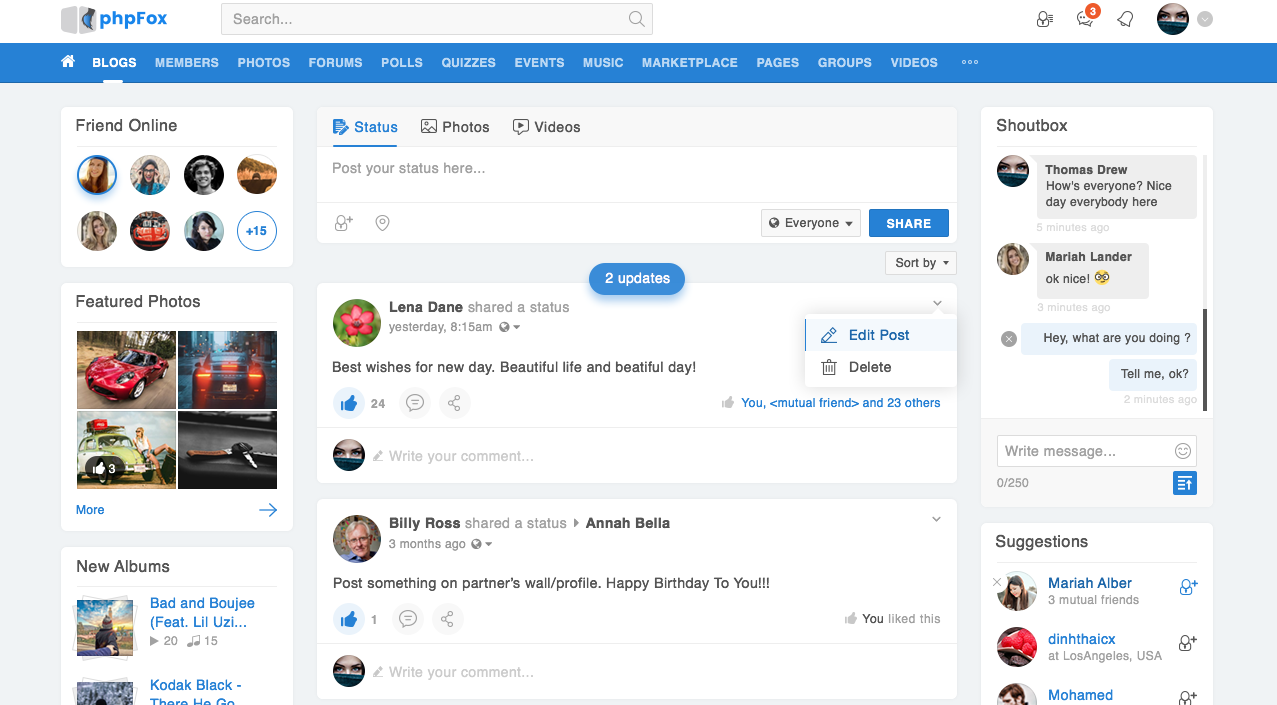The screenshot displays a website that prominently features "phpFox" at the top, possibly indicating it is built on or utilizing the phpFox platform. The interface includes a search bar situated in the top left corner. On the right side, there is an image of a woman wearing a mask, likely for COVID-19, with her eyes clearly visible. Adjacent to this image are icons indicating she has three unread messages. Below the header is a small blue navigation bar containing links labeled: Blogs, Home, Members, Photos, Forums, Polls, Quizzes, Events, Music, Marketplace, Pages, Groups, and Videos.

The overall layout bears a striking resemblance to Facebook, with a predominantly blue color scheme, although the shade is slightly lighter than Facebook's. The homepage features a feed displaying various posts from users. On the right side of the page, there's a section labeled "Shoutbox," where users appear to be engaged in a casual conversation. For example, a user named Thomas Drew has posted a message saying, "How's everyone? Nice day everybody here," to which another user, Mariah, responded with, "Okay, nice," accompanied by a whimsical-looking emoji.